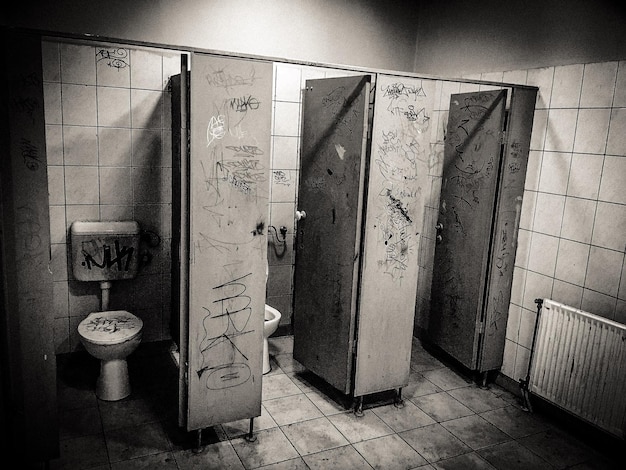The image is a haunting black and white photograph of an old, decrepit public bathroom, filled with a dismal and neglected atmosphere. The bathroom features three stalls with metal doors, all of which are swung open to reveal the filthy interiors. The floors and walls are tiled, though the tiles look grimy and coated with years of dirt, adding to the overall sense of decay. Practically every visible surface is covered in graffiti, as if the bathroom has been overtaken by vandals over the years. The graffiti is not artistic but rather a chaotic mess of scribbles and tags, often hinting at possible gang affiliations.

Each stall showcases its fair share of defilement; the toilets, with their tanks mounted on the wall, are marred with graffiti on both the lids and tanks. Specifically, the leftmost stall displays a closed toilet lid plastered with markings, while the middle stall reveals the edge of a toilet bowl with the lid up. The right stall's door is open, yet its toilet remains out of view. A rusty, dilapidated radiator clings to the right wall, further emphasizing the long-forgotten state of the facility. The lighting in the photograph is dim, and the grayscale color scheme, with a slight sepia tone, accentuates the dreariness of the scene, invoking a bleak, almost post-apocalyptic ambiance.